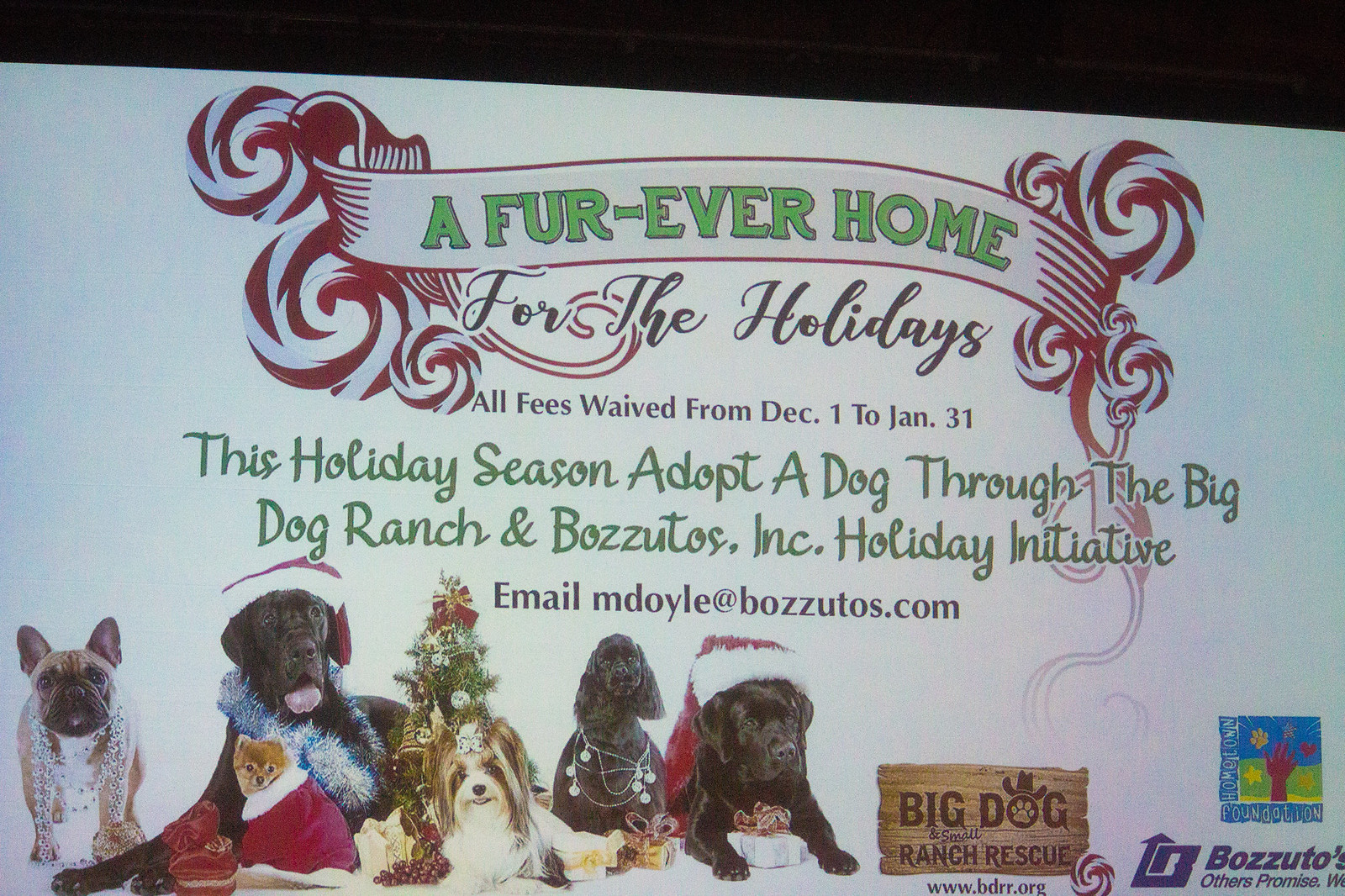This holiday adoption flyer has a festive theme and a white background, featuring a vibrant red and white animated sleigh design at the top. Centered within this design, a white ribbon displays the message in green text: "A Fur-Ever Home." Directly below, in elegant black script, it reads, "For the Holidays." Another black serif line underneath announces, "All Fees Waived from December 1 to January 31." Following this, in green script, it states, "This Holiday Season Adopt-A-Dog Through the Big Dog Ranch and Bozutos, Inc. Holiday Initiative." For more information, it lists an email address, "mdoyle@bozutos.com."

Below the text, on the left, are charming photos of around six dogs, engagingly set in a Christmas atmosphere. These include breeds such as a French Bulldog, a grey dog that could be a Weimaraner, a tiny orange kitten in a Santa jacket, a Yorkie or Lhasa Apso with a bow, a black or brown Cocker Spaniel adorned with holiday lights, and a black Labrador puppy sporting a Santa hat beside a wrapped gift. A small decorated Christmas tree is part of this festive setup. Adjacent to the dog images is a light brown rectangle with the logo "Big Dog Ranch Rescue," featuring a cowboy hat over the 'O'. At the bottom right, additional branding includes a blue square with a red figure, an arrow pointing upward logo, and the bold italicized name, "Bozutos."